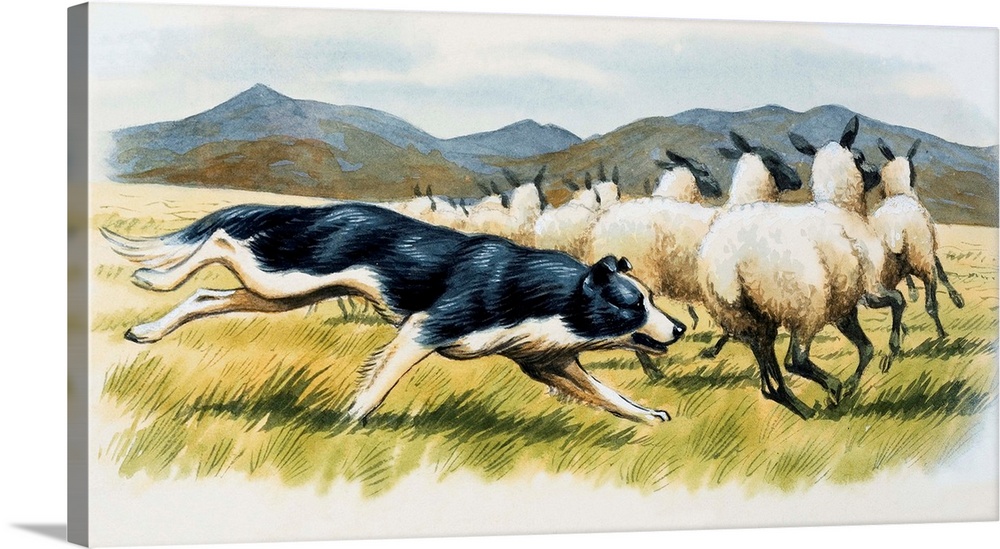This dynamic painting vividly captures a herding dog energetically chasing a flock of sheep. The dog, possibly an Australian sheepdog, is portrayed with striking black and white fur. Its elongated rear legs are airborne while its front legs maintain a sprinting stance on lush green grass. The dog’s back and the area over one of its eyes are cloaked in shiny black fur, while its snout, legs, and the base of its tail are white, with hints of brown on the left legs potentially depicting shadows. The dog's fur pattern with the black resembling a blanket draped over its back accentuates its sleek physique and motion.

To the right of the dog, approximately ten sheep are depicted in full flight, their fluffy white bodies with contrasting black faces, ears, and legs captured in mid-run. The artist masterfully conveys a sense of urgency and motion as the sheep flee from the dog, their limbs also elongated in motion.

In the background, a serene landscape unfolds with grayish-brown mountains under a predominantly light blue sky, adding depth to the scene. The painting, devoid of any artist's mark or signature, presents a vivid and dynamic representation of a classic pastoral activity.